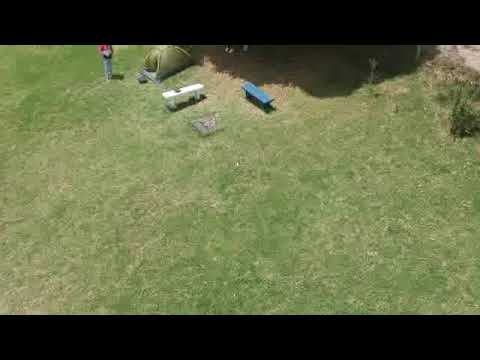This image appears to be a downward, slightly angled aerial view of a grassy field. The photograph is captured with black borders at the top and bottom, resembling a widescreen format. The overall image is blurry and pixelated, making finer details difficult to discern. However, noticeable elements include two benches in the scene: one blue bench towards the top middle, angled downward with the right side pointing southeast, and another white bench positioned on the left side, angled southwest. To the left of these benches, there is a person facing toward the camera. The individual, who appears to be wearing a red shirt and blue or gray pants, is positioned next to something that could be a small green tent. Additionally, there is a shadow to the right which may indicate the presence of a tree. The image suggests a possible drone perspective or an elevated vantage point for the photograph.